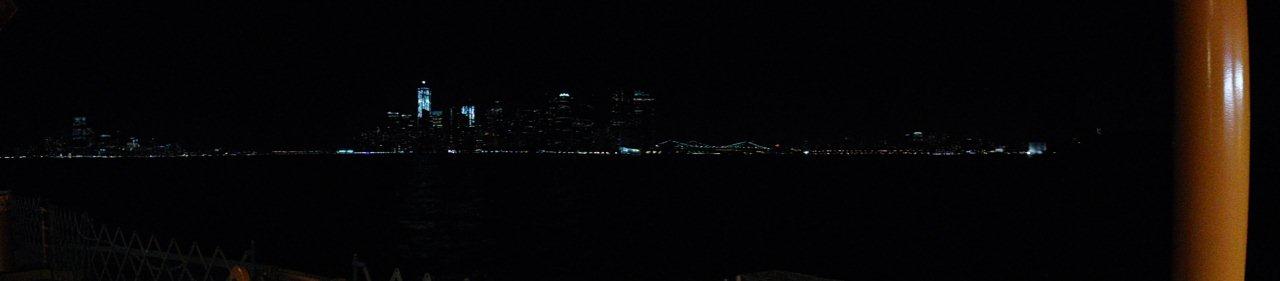Captured from across a dark, seemingly tranquil body of water, this nighttime image showcases a luminous cityscape, potentially New York City, set against a pitch-black sky. Dominating the scene are two brightly illuminated skyscrapers on the opposite shore. The left skyscraper, taller and imposing, is adorned with aqua blue lights, likely the One World Trade Center. To its right, albeit a number of blocks away and appearing closer due to depth perception, stands another tall building emitting a similar blue glow. Scattered white lights trace the shoreline, enhancing the urban silhouette. In the foreground on the left, a brown circular pole, possibly indicating the photographer's position on a ferry or boat, catches some reflected light, subtly outlining its presence. The expansive view hints at more city lights stretching towards the horizon, interspersed with shorter lit-up buildings and a bridge on the far right, all contributing to the captivating allure of the nocturnal metropolis.